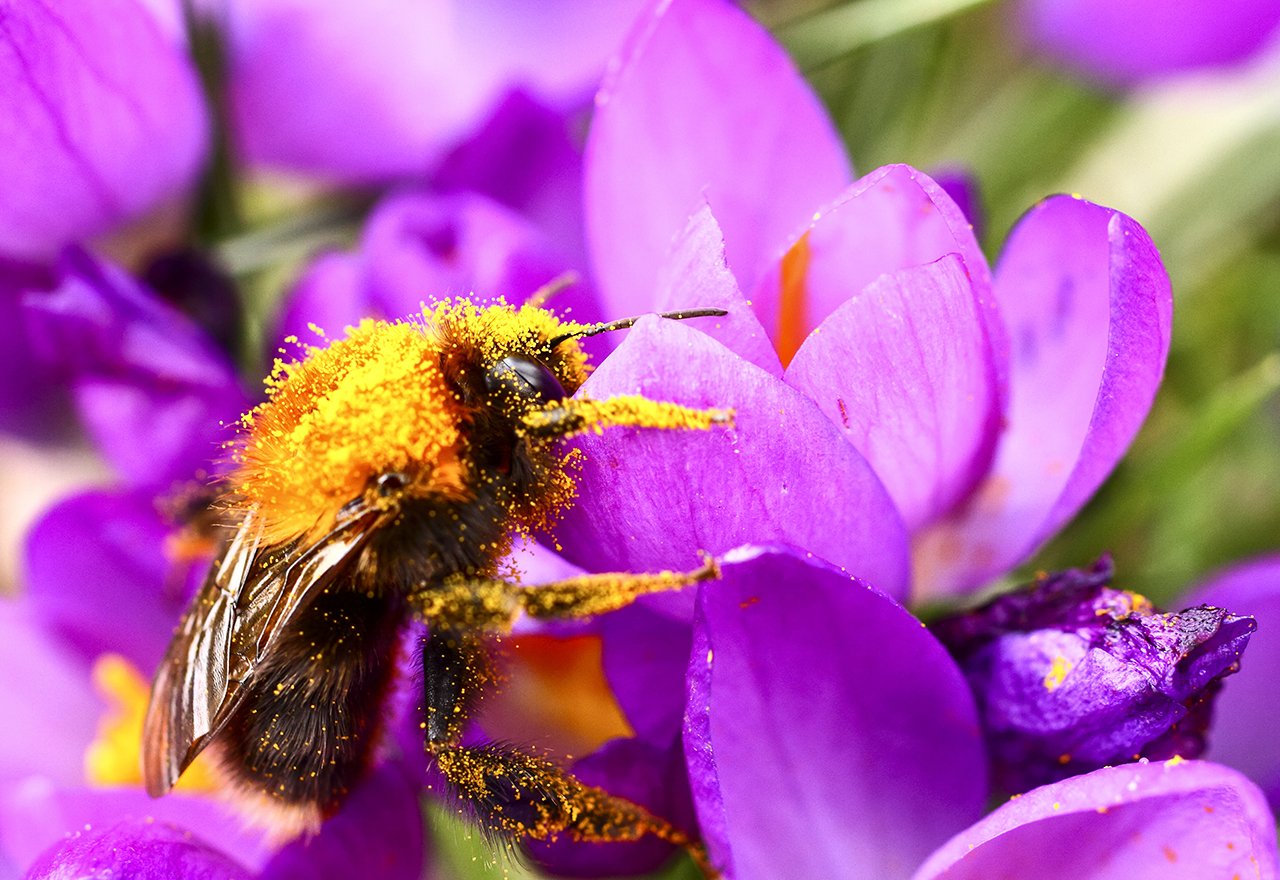The close-up photo captures a dark-bodied insect with a yellow back, which appears to be a bumblebee, clinging to the vibrant petals of a purple flower. The bee is heavily dusted with yellow pollen, which is visible on its back, head, and legs. Its wings are folded tightly against its body as it navigates through the dense pollen. The well-lit photograph highlights the varying shades of the purple flower petals, ranging from light to dark depending on the light's angle. In the blurred background, additional purple flowers and lush green stems and leaves create a vibrant, natural setting. The scene suggests the bee might be struggling slightly due to the heavy pollen load, adding a dynamic aspect to the image.